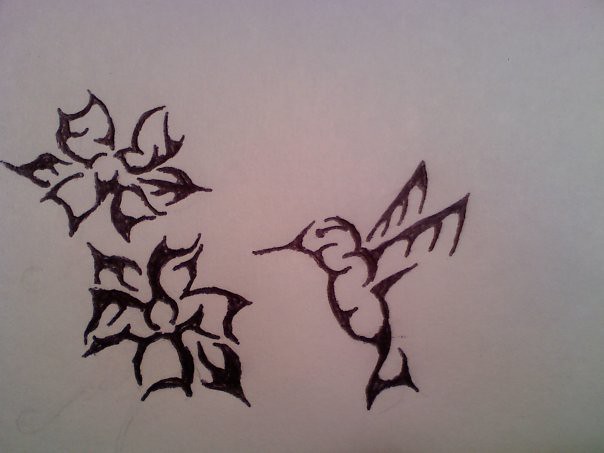This ink drawing on a plain white sketch paper depicts a delicate scene of two flowers and a hummingbird. The flowers, positioned on the left side of the image, are stacked vertically, one above the other, with intricate outlines hinting at their petals and stems. To the right, a intricately outlined hummingbird is captured in mid-flight. The bird features an elongated beak extended towards the left, as if aiming to sip nectar from the flowers. Its body leads to a unique, Z-shaped tail that zigzags down to the left, up again, and finally points upward. The hummingbird's wings stretch straight out, each adorned with three curved lines and ending with a sharp, spiked feature pointing to the right. The entire illustration remains in monochrome, using only the pen's ink for contours and details, showcasing the artist's careful attention to form and movement.